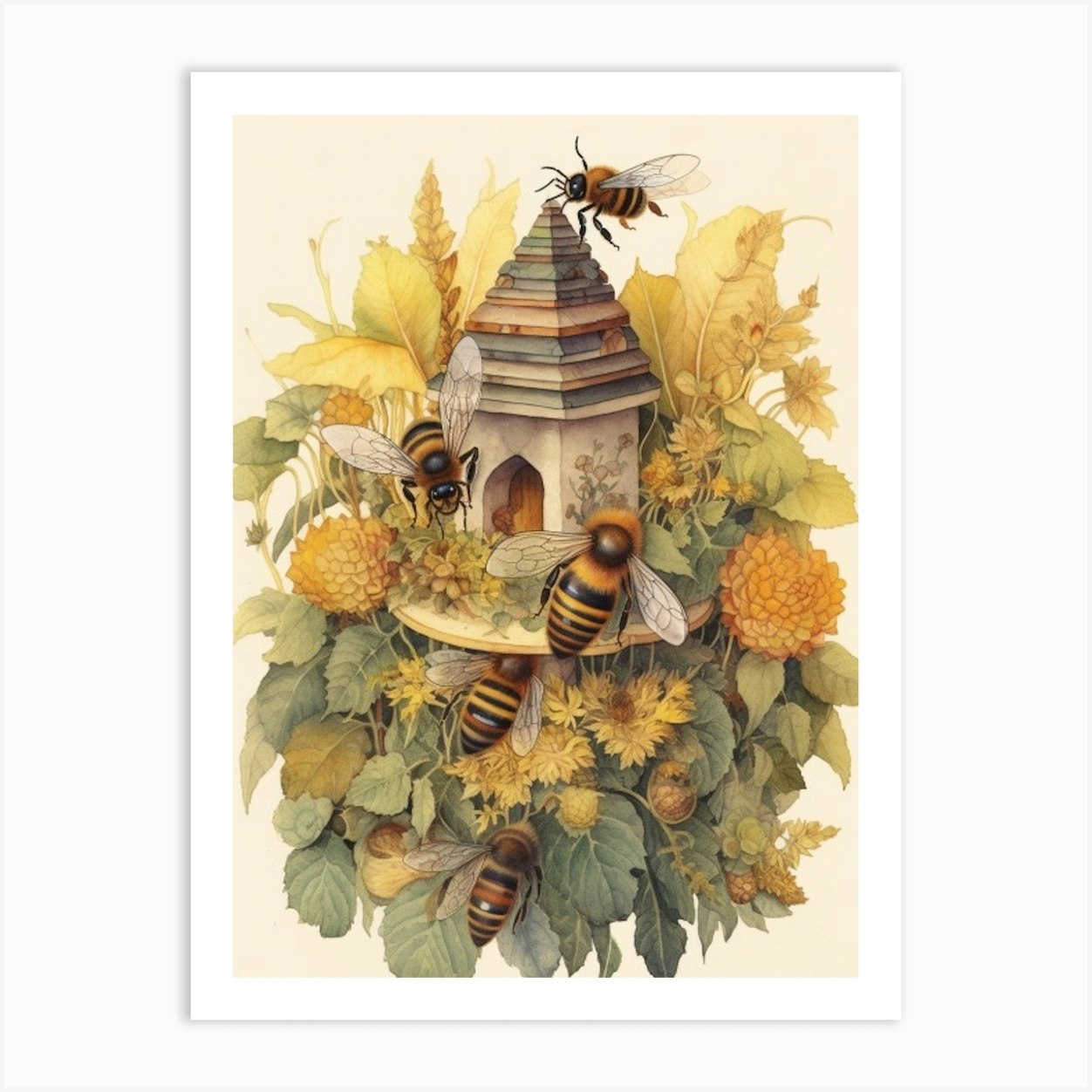This detailed illustration resembles a whimsical bird feeder transformed into a charming bee house. The structure, standing vertically, has a rectangular form with a pointed, multi-layer triangular roof adorned with hints of red, blue, and green, though the overall color palette is more subdued and hued down, giving it a less vibrant appearance. The central structure features a small wooden door, suggesting a miniature home or even a fairy house.

Surrounding this bee house is a dynamic scene of green and yellow leaves interspersed with orange and yellow flowers, likely mums or marigolds, enhancing the fanciful nature of the image. Five stylized bees with orange and black bodies are scattered across the composition, concentrated mostly around the middle of the structure. One bee perches at the top, another on the side of the building, and the remaining bees are positioned more towards the bottom, creating a sense of movement and liveliness.

The illustration is set against a beige background, framed by a white border, which makes the central elements stand out. With no people or text present, the image focuses solely on the enchanting interplay between the bees, the bee house, and the floral surroundings, encapsulating a whimsical, yet detailed portrayal of a serene natural habitat.